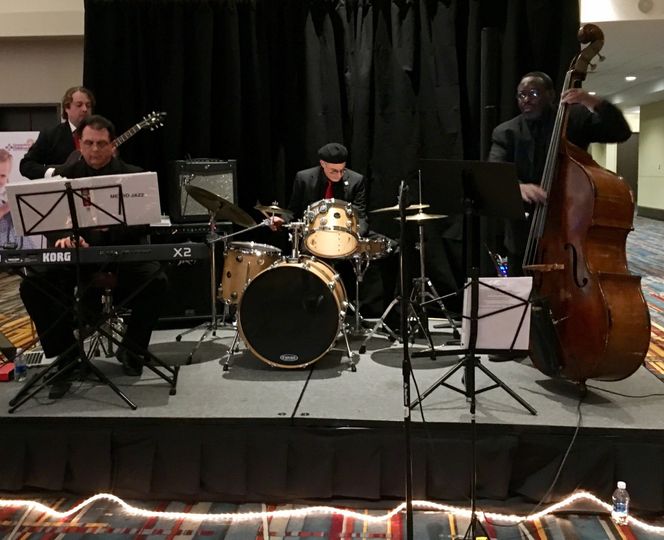A band of four musicians is performing on a small, slightly elevated stage, approximately one and a half to two feet off the ground, beneath a black curtain. The stage is adorned with rope lighting and scattered with water bottles. Each musician is dressed in black suits, with varying accents; one wears a black beret and glasses, while two bear red ties. Central to the stage, the drummer, a white man, focuses on his yellowish drum set with a prominent black snare. To his right stands a tall African American man in glasses, playing a large stringed instrument likely an upright bass, often mistaken for a cello. To the far right, a white male keyboardist intently studies his sheet music, one hand poised on his Korg keyboard. Behind him, slightly obscured, another white man holds an electric guitar. The ambiance suggests a formal setting, possibly a convention or smaller event, highlighted by the rental-like fabric stage covering and presence of amps and music stands. They're immersed in their musical set, creating an atmosphere of professional performance.